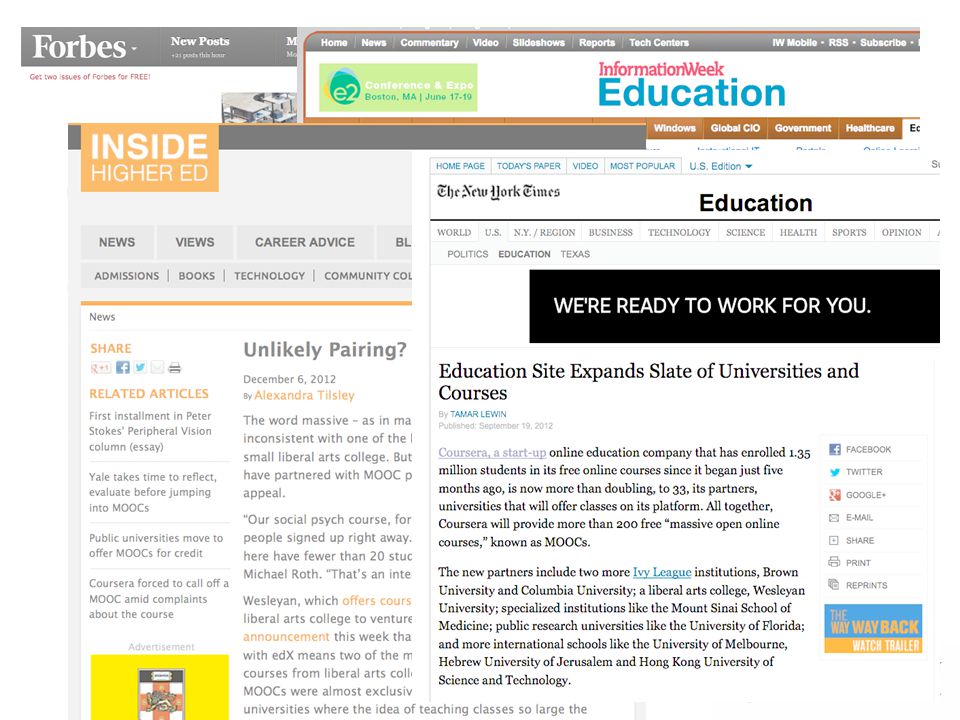The image is a collage of various text elements and logos from different educational and informational sources, positioned on a visually busy layout.

- In the upper left corner, "Forbes" is written in white text with "New Posts" also in white, situated just beside it.
- Towards the right, "Information Week, Education" appears, with "Education" highlighted in blue text.
- "Inside Higher ED" is displayed within an orange square.
- Further to the right, "The New York Times" is mentioned in its distinctive font style, with the word "Education" in black, enclosed within a black rectangle.
- Beneath this, a bold statement reads, "We're ready to work for you," followed by "Education site expands slate of universities and courses."
- The body of the text includes two informational paragraphs, where the term "Ivy League" in the second paragraph stands out, highlighted in blue and underlined.
- On the far right, there are various sharing options, including icons for Facebook, Twitter, Google+, Email, Share, Print, and Repeat.
- A small blue square saying "The Way Back" is positioned below the sharing icons.
- Lastly, at the bottom of the image, under a yellow rectangle, there is a prompt that reads "Watch Trailer" in small white text.

Overall, the image integrates multiple sources and emphasizes educational content, providing various interactive elements and highlights for the viewer.